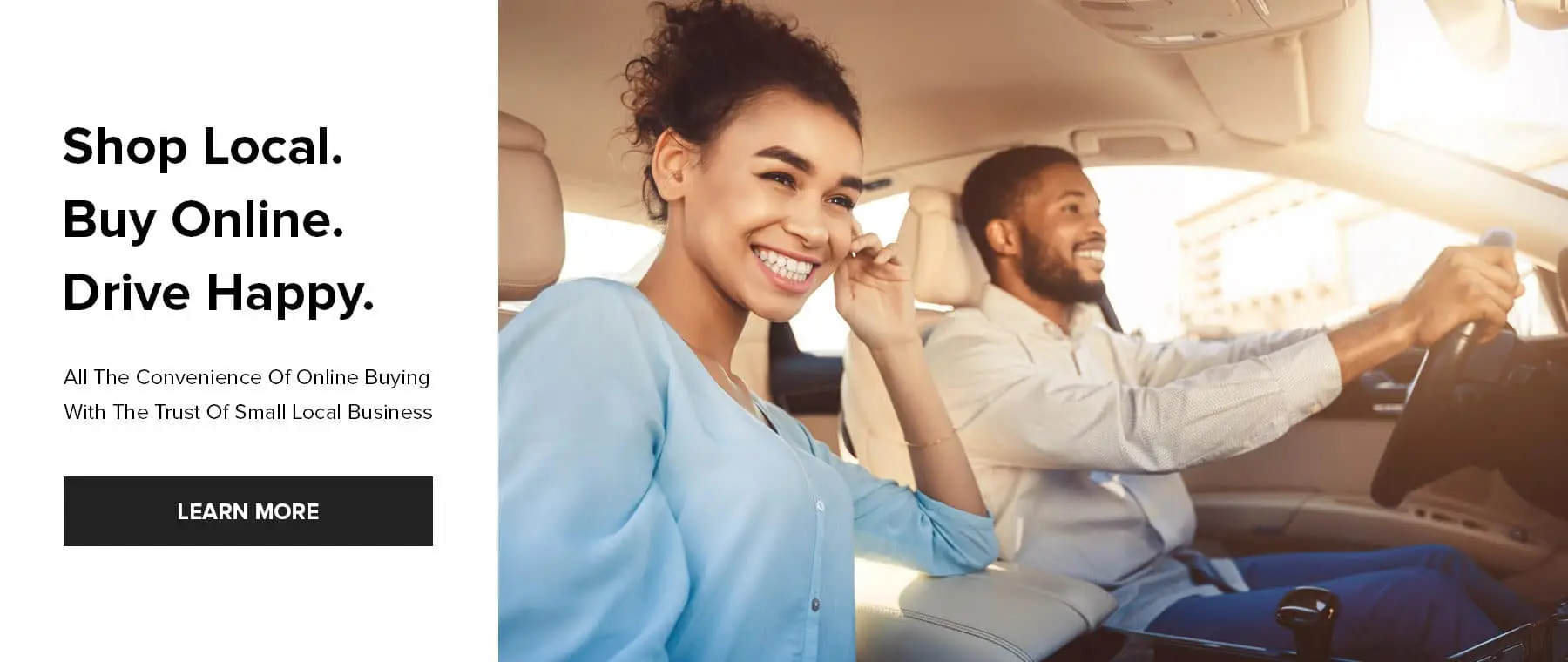To the left of the image, there is a rectangle with three lines of bold black text: "Shop Local. Buy Online. Drive Happy." Beneath this, in smaller black letters, it reads, "All the convenience of online buying with the trust of small local business." Below this text is a black rectangle featuring the words "Learn More" in white. 

The photo depicts a happy couple sitting inside a car. The driver is a black male, wearing a white or cream-colored long-sleeve shirt, paired with blue jeans. He has a beard and a mustache, and his head rests against the light tan headrest. His hands are on the steering wheel, and he is smiling. Beside him, a black female is seated, wearing a light blue shirt. She is smiling brightly, with her elbow resting on the center console and her hand gently touching her left cheek. Her hair is pulled back, revealing her joyful expression. The interior of the car is a soft beige, and through the driver's side window, the exterior of a building is visible.